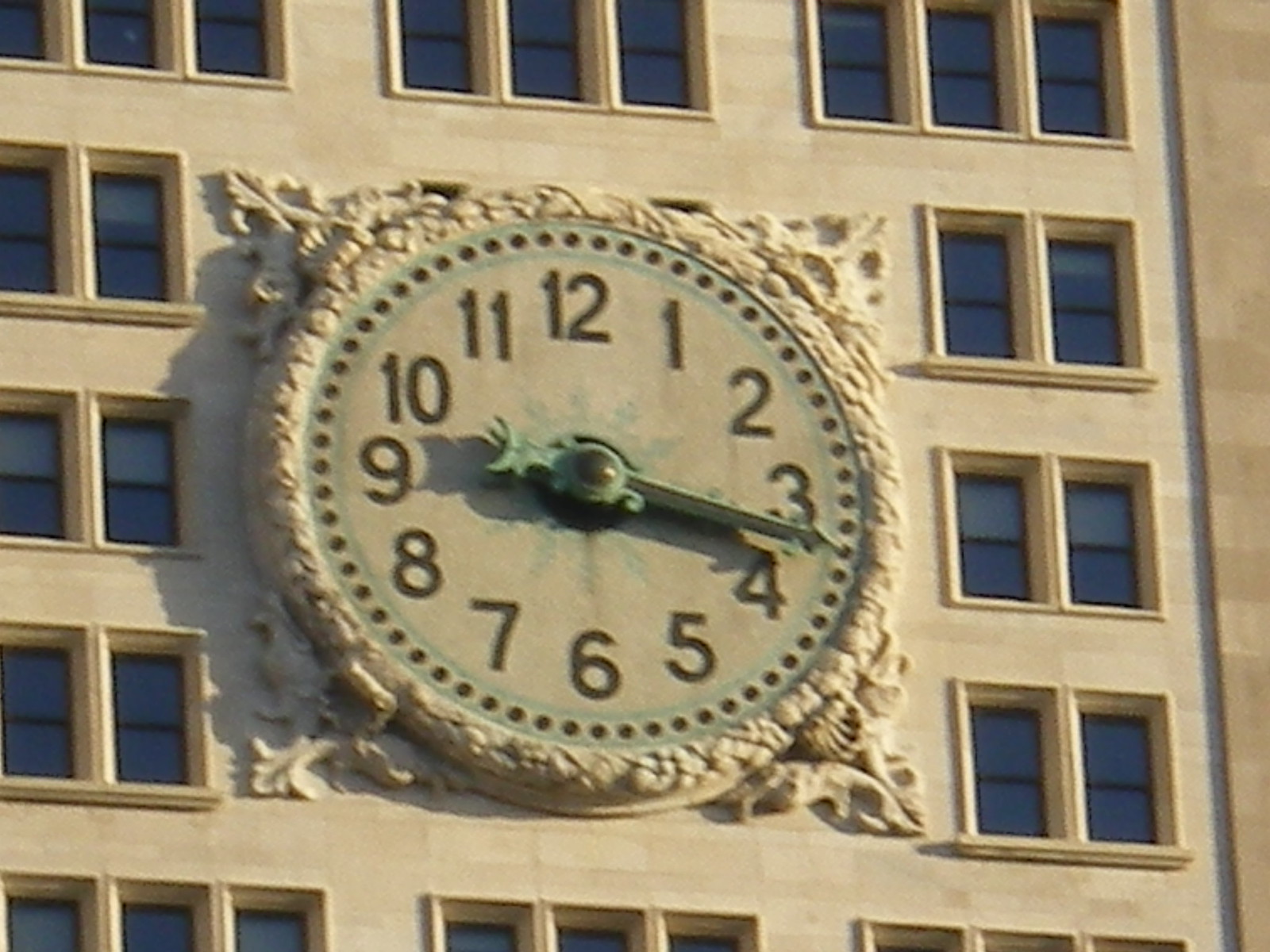This color photograph is a detailed close-up of a large, ornate clock mounted on the exterior wall of a building. The clock itself is round with an elaborate carved border in a light hue, possibly white or cream, extending at its four corners to form a square-like shape with Victorian-era styling. The face of the clock is a pale, weathered green, interspersed with streaks of darker green, and encircled by two green cycling rings. Within these rings, there is a row of small black dots marking the seconds. The clock displays black numerals ranging from 1 to 12 and features ornate green hands. The minute hand points between 3 and 4, while the hour hand is positioned near 10, though there's a slight shadow causing some visual ambiguity. The clock is mounted against a beige, chalky building adorned with multiple sets of windows. These windows are grouped in sets of 2 or 3, featuring dark blue panes, with some being placed above, below, and to the sides of the clock. Light casts shadows to the left, suggesting the sunlight is coming from the right side of the image.